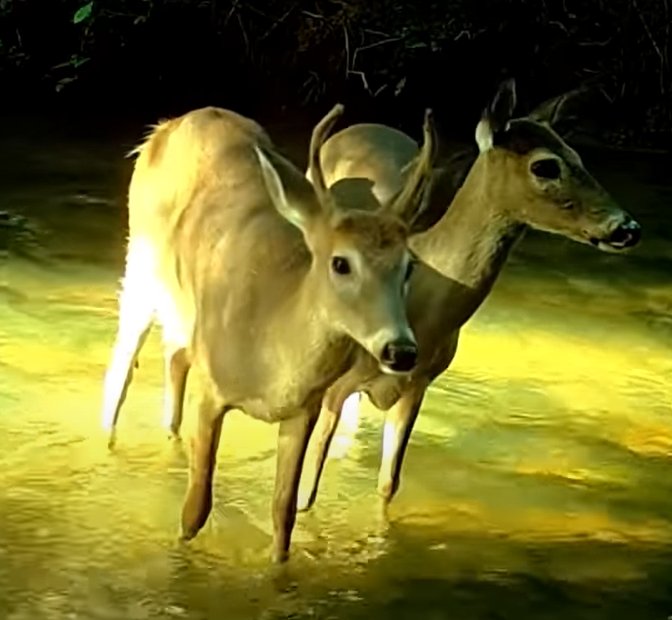A night vision image captures two young deer standing in shallow water, their light brown coats and dark eyes stark against the eerie, green-tinted surroundings. The image quality is pixelated, hinting it was taken with some night vision technology. Both deer appear startled, their expressions frozen in surprise as they look in different directions – the one on the left facing the camera with small antlers illuminated by a bright light, while the other gazes off to the side. Faint tree branches obscure the dark background, adding to the mysterious and somewhat unsettling atmosphere. The water, tinted green and barely reaching above their hooves, adds an extra layer of intrigue to this nocturnal scene.